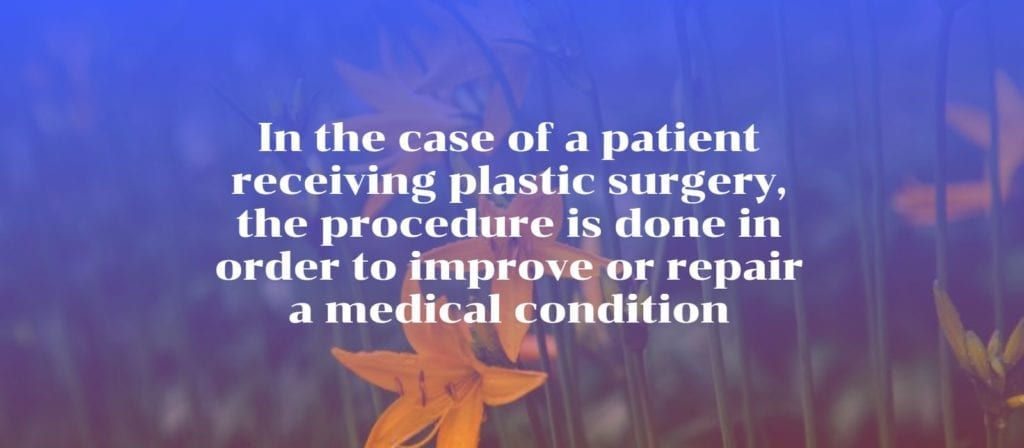The image features a slightly blurry background filled with green stalks of wild yellow flowers, some of which extend beyond the image's top edge. Prominently, there are three yellow flowers in the middle and one flower on the right side. The overall background hue appears predominantly blue and purple, giving the scene a serene feel. Overlaying this botanical backdrop, white-centered text spanning five rows reads, "In the case of a patient receiving plastic surgery, the procedure is done in order to improve or repair a medical condition." The clear and concise text, with each line beginning with an uppercase letter, suggests a context of medical information, likely for a poster in a doctor's office or a hospital setting.